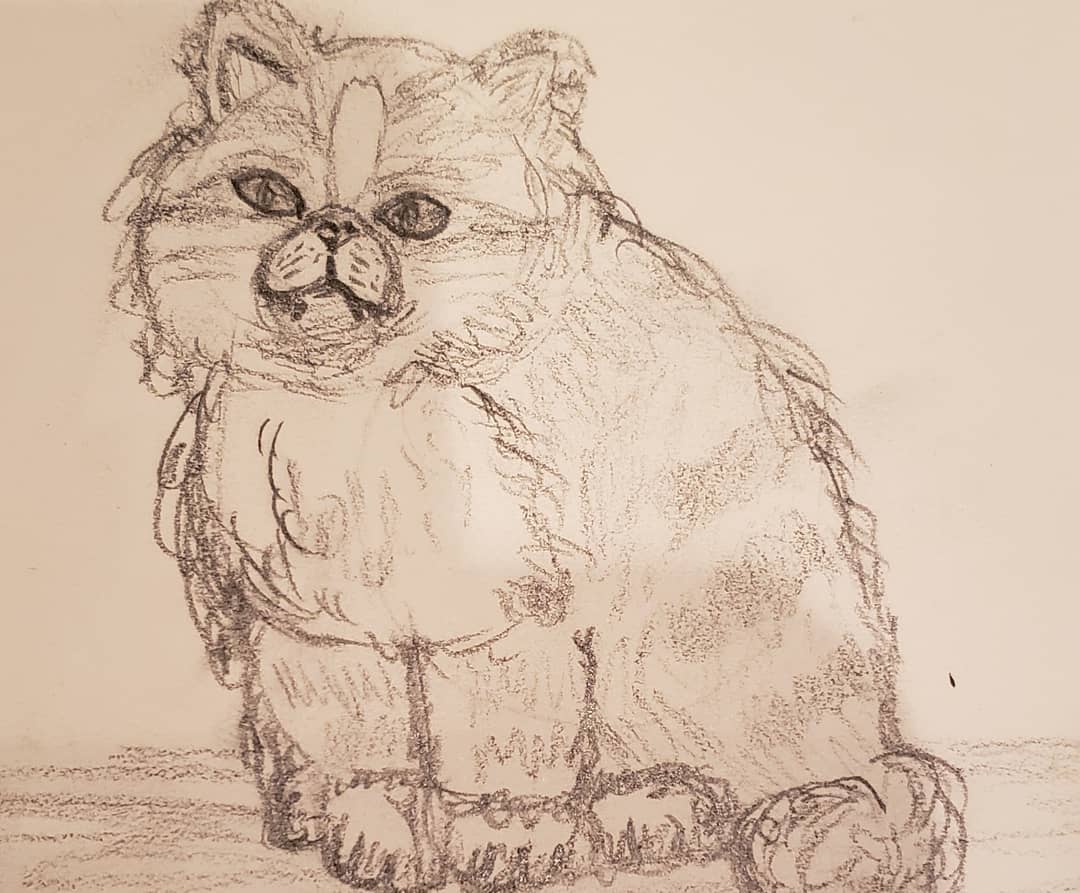This image is a detailed photograph of a hand-drawn sketch of a cat on a light tan, antique-looking piece of paper. The drawing appears to be created using possibly a single crayon, pastel, or colored pencil. The cat, sitting on its bottom with front paws extended in front, is depicted with a chubby, healthy appearance and a fluffy texture achieved by using curly, fluffy shapes instead of a traditional outline. The artist emphasized the facial features by deepening the color on the eyes and nose, giving the cat a serious, almost slightly angry expression. The cat's ears are pointed, with the right ear appearing darker. The cat's tail is fluffy, and the sketch features broad brush stroke-like stripes, particularly around the head where an opening is left to suggest a white forehead. Notably, the cat is missing whiskers, and the overall background remains the original beige tone of the paper.